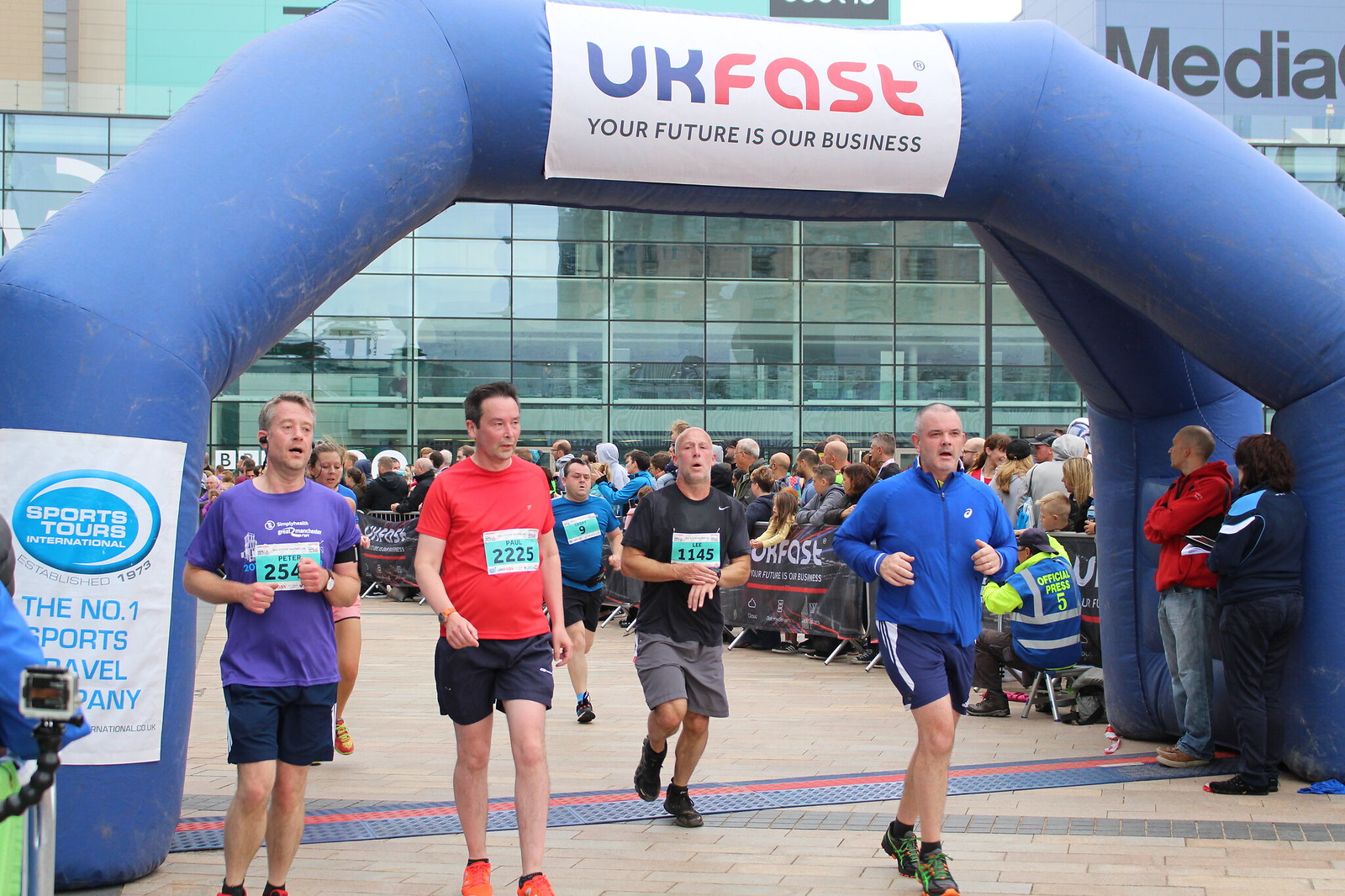In the picture, we see four men finishing a race under a large blue inflatable arch, which serves as the finish line. The arch, positioned in the middle of a brick-floored street, reads "META" on the right and partially displays the words "sports tours" on the left, though some of the text is obscured by an arm. The runners are dressed in shorts, t-shirts, and other sporting gear, with numbers pinned to their chests. One man is just crossing the finish line, while another follows closely behind. A crowd of spectators stands behind barriers on both sides of the street, watching the racers intently. In the background, there is a large, glass-windowed building, with several other structures visible further behind. The event appears to be happening outdoors, in the middle of the day, characterized by contrasting bright and dark colors, including shades of blue, red, purple, lime green, black, and white.